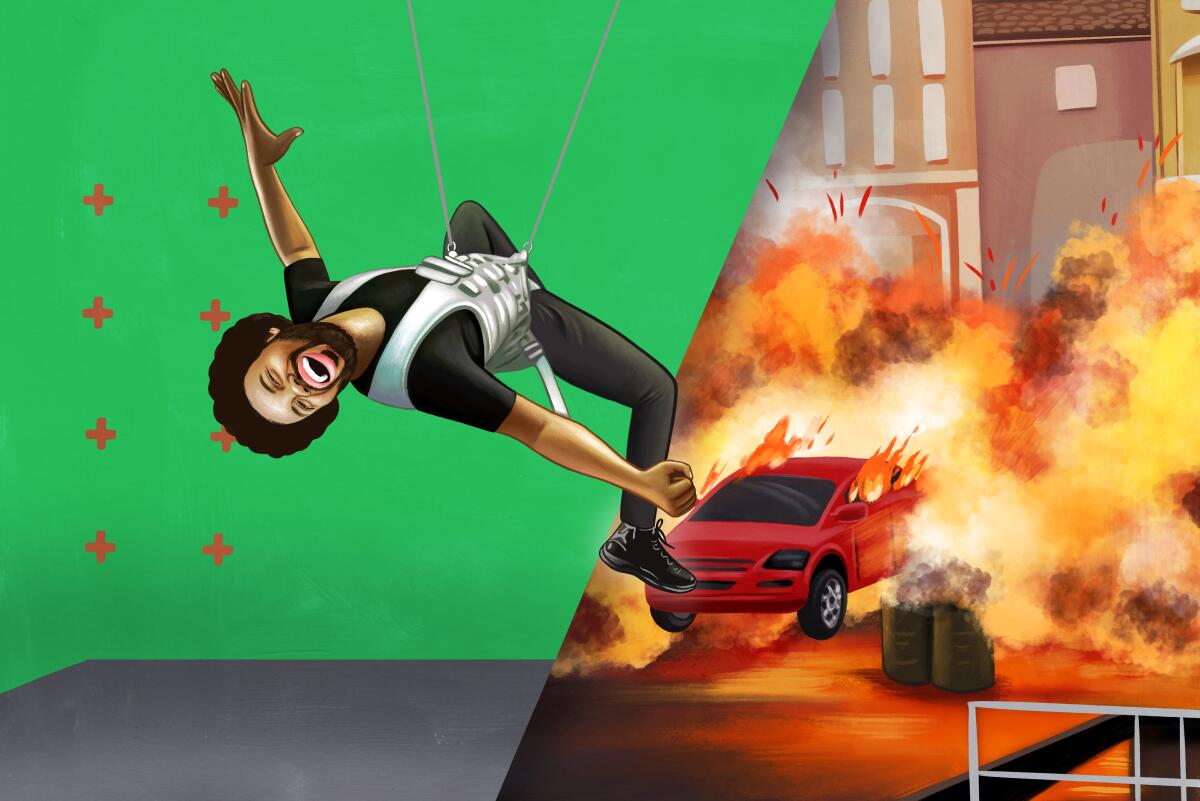The image appears to be a computer-generated artwork divided into two distinct parts. The left side depicts an indoor setting with a green background and a gray floor, adorned with eight red crosses arranged in two rows. A Black African-American man, wearing a silver vest over a black t-shirt and black pants, is suspended from the ceiling by metal wires attached to his waist. He hangs with his stomach facing upward, arms stretched wide, head tilted back with eyes squinted shut, and a wide, joyous smile on his face, giving the impression that he is floating and enjoying himself. The right side portrays an outdoor scene amid chaos, featuring a red sports car seemingly launched into the air, trailing flames and smoke. The car's windows are ablaze, and surrounding barrels and trash cans are also on fire. In the background, a tall building looms behind the thick smoke and fire, adding to the sense of destruction and mayhem.